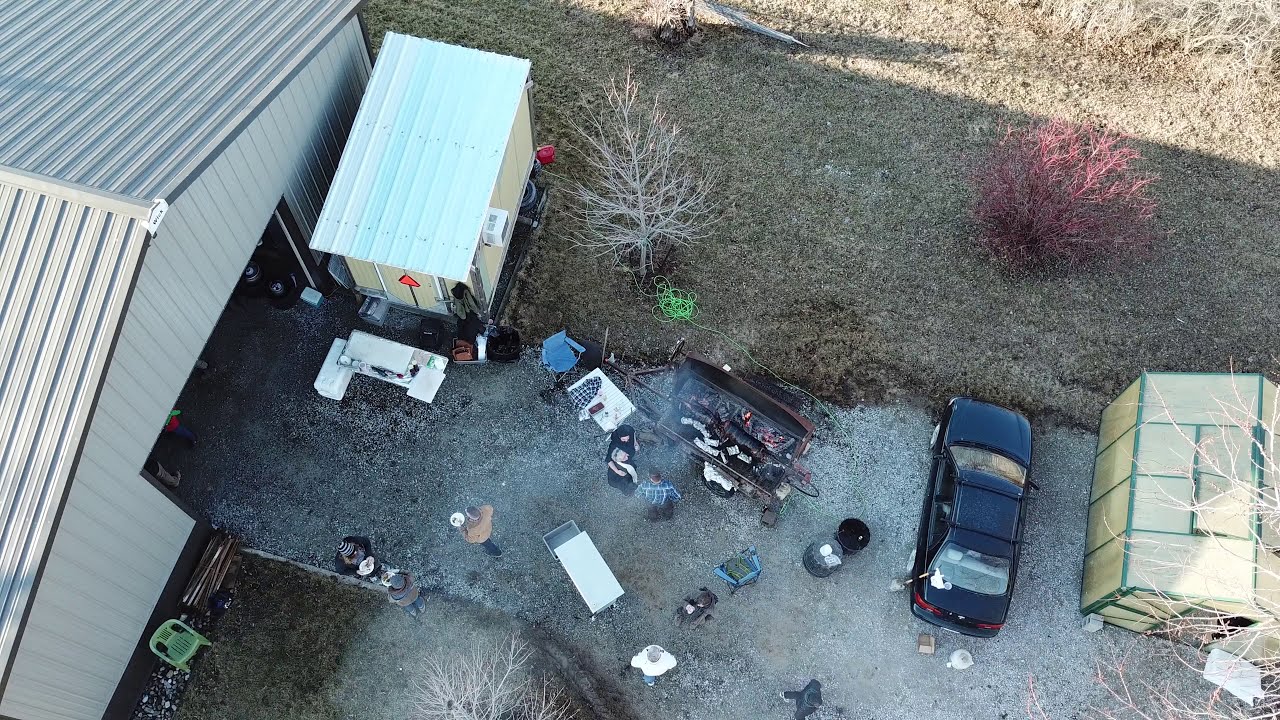From an aerial drone perspective, the image showcases a small gathering centered around a large grill where several people appear to be barbecuing a variety of meats. In the middle ground, there is a metal, barn-like structure with an open door. This white, metal-roofed enclosure is situated on the left-hand side of the image. Adjacent to it is a smaller, shed-like structure. Towards the bottom right corner, a dark blue or black car is parked beside a yellowish tent with green accents. The concrete pavement in the lower part of the image features scattered folding chairs and furniture, indicative of a casual get-together. Surrounding the scene, the landscape mostly consists of dried grass and dirt with minimal greenery, and a couple of bushes—one notably with pinkish-red leaves. You can also spot a dead tree near the parked car. The overall atmosphere suggests a cookout event, with attendees holding white plates likely filled with barbecued food.